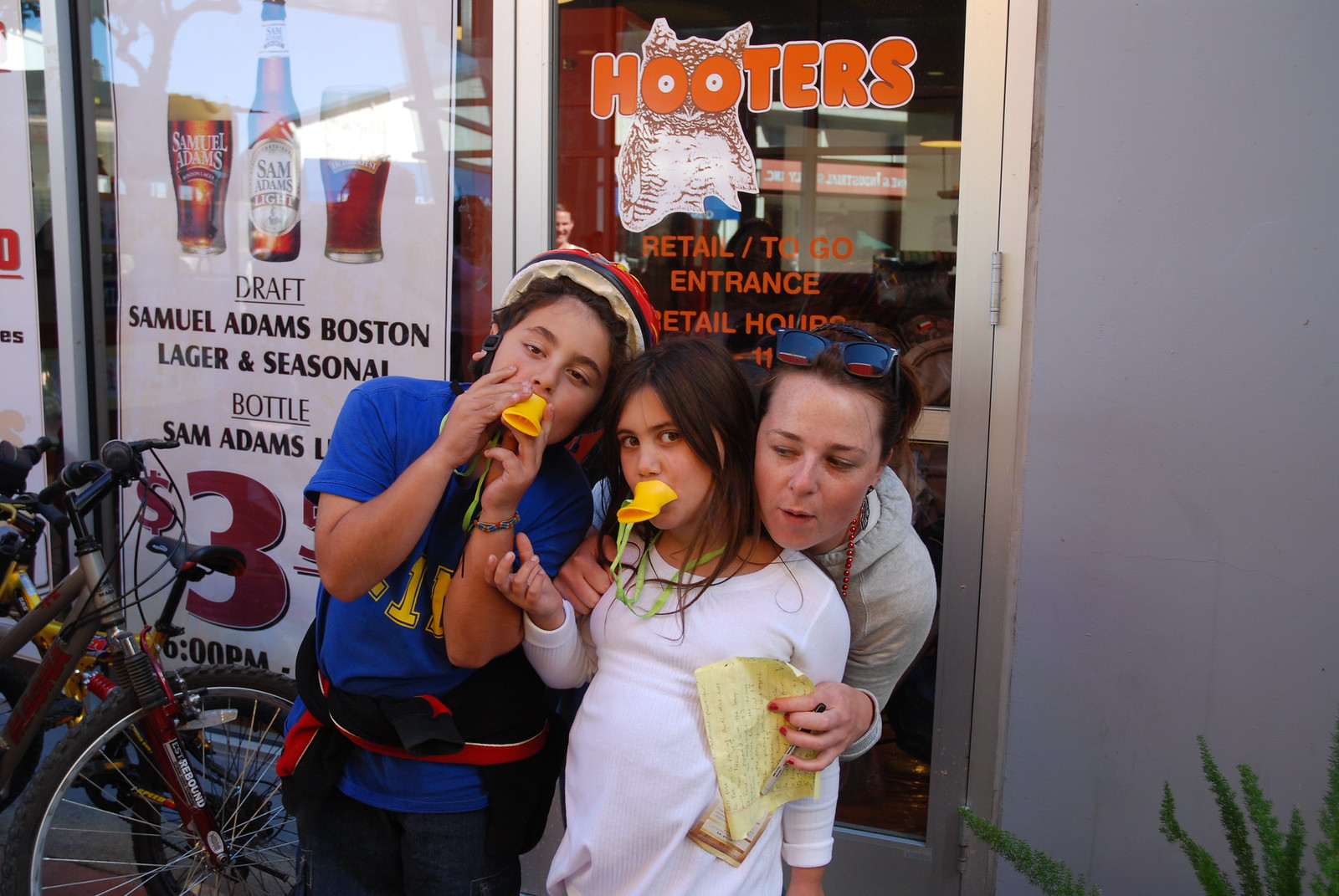This photograph captures a lively scene outside a Hooters restaurant. Prominently positioned in front of the door, which features the iconic Hooters owl logo with big orange eyes and white irises forming the "O"s, are three people. On the left, a girl in a red bicycle helmet and a blue t-shirt with red lettering is blowing into a yellow whistle or balloon. She has a brown and red sweatshirt wrapped around her waist. Beside her, a younger girl in a pink long-sleeve shirt is also blowing a yellow whistle toward the camera. Behind them, an adult woman is kneeling, bending over the younger girl's shoulder while holding a yellow piece of paper and looking down at it. She is steadying the younger girl by holding onto her shoulders. To the left of the image, two bicycles are partially visible. The scene is set against a mix of gray wall to the right and the busy entrance of the Hooters establishment, adding a vibrant and dynamic backdrop to the energetic interaction in the foreground.